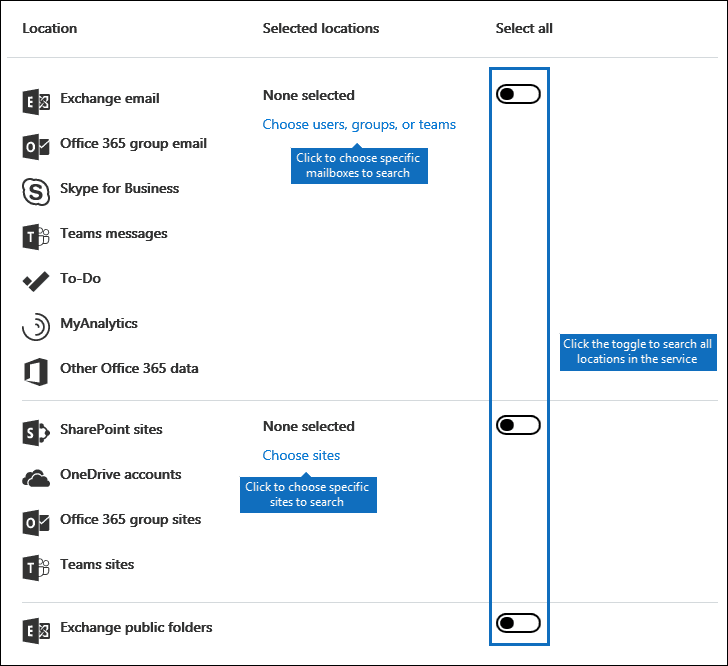The image displays a software interface for selecting items on a PC, presented against a white background. The interface is surrounded by a thin pixel border at the top edge. At the top of the menu, there are options labeled "Location," "Selected Locations," and "Select All." In the "Location" section on the left, items are listed with corresponding icons: Exchange Mail (Exchange logo), Office 365 Group Email (Office 365 logo), Skype (S logo), Skype for Business (S for Skype), Teams Messages (T for Teams), To Do tasks (check mark icon), My Analytics (circular icon), Other Office 365 Data, SharePoint Sites, OneDrive Accounts, Office 365 Group Sites, Team Sites, Exchange, and Public Folders.

The "Selected Locations" section indicates "None selected." Instructions are overlaid with a blue field, advising to "Choose user groups or teams, click to choose specific mailboxes or search." 

Under "Other Office 365 Data," a horizontal line stretches across the width of the interface. Next to "SharePoint," it states "None selected," with a reminder to "Choose sites again, click to choose specific sites or search."

On the right side of the rectangular, highlighted area, there is an option to "Click to toggle the search or view all locations in the service." Toggle buttons appear next to Exchange Mail, SharePoint, and Exchange Public Folders, allowing users to switch the selection status within this category.